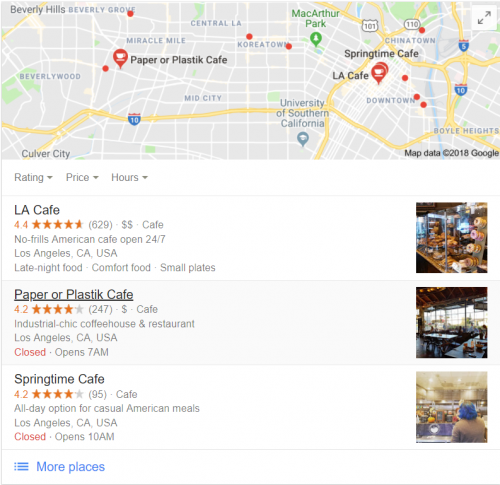This image is a screenshot presumably from a map or restaurant-review application, evident from the map data credited to Google (2018) at the top corner. The map displayed focuses on various neighborhoods in Los Angeles, including Beverly Wood, Beverly Hills, Central LA, and Koreatown. Prominent in the map are three larger markers with coffee cup icons, indicating café locations: Paper or Plastic Cafe, LA Cafe, and Springtime Cafe. 

The "Paper or Plastic Cafe" seems to be the selected item, highlighted with a black underline. Below the map, detailed information is available for these three cafés, including their names, types of food served, reviews, locations in Los Angeles, and operating hours. Additionally, each cafe listing is accompanied by a thumbnail image on the right-hand side. 

Overall, the image provides a concise overview of café options in the specified Los Angeles neighborhoods, integrating essential details and visual markers for easy navigation and comparison.